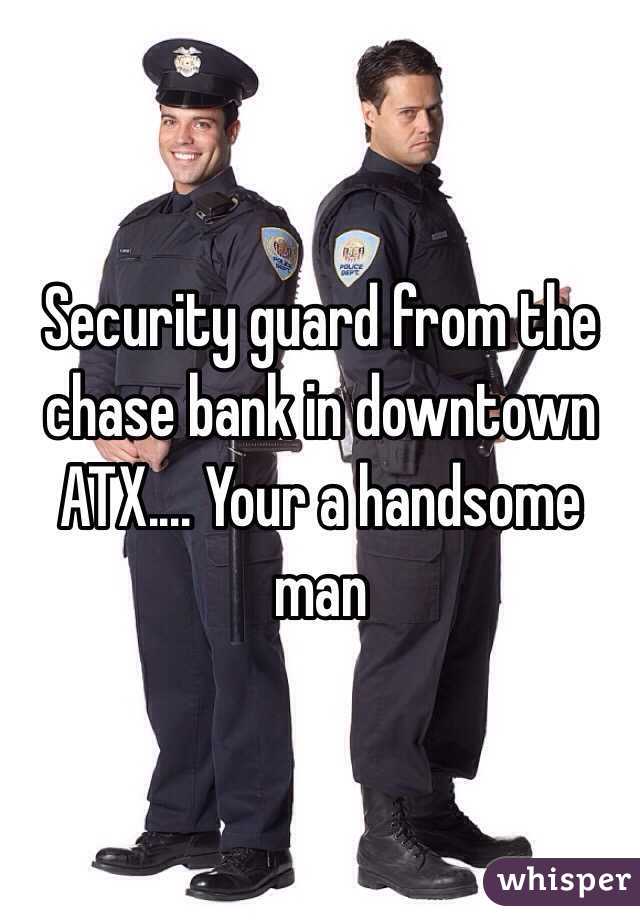In this image, two security guards standing shoulder-to-shoulder appear distinctly contrasting yet uniform in their presentation. Dressed in dark blue uniforms with patches labeled "Police Department" on their shoulders, the guard on the left dons a black uniform hat with a centered badge and displays a wide smile, revealing his teeth. His hands rest on his belt, giving a relaxed demeanor. In contrast, the guard on the right stands seriously, devoid of any smile, and is hatless, showcasing his short brown hair. He clutches a baton in his hands, reinforcing his stern appearance. Both guards are equipped with black combat-style boots. Overlaying the center of the image, white text reads: "Security guard from the Chase Bank in downtown ATX... You're a handsome man," spread across four centered lines. At the bottom right corner, the word "Whisper" is inscribed in white text against a plain background.